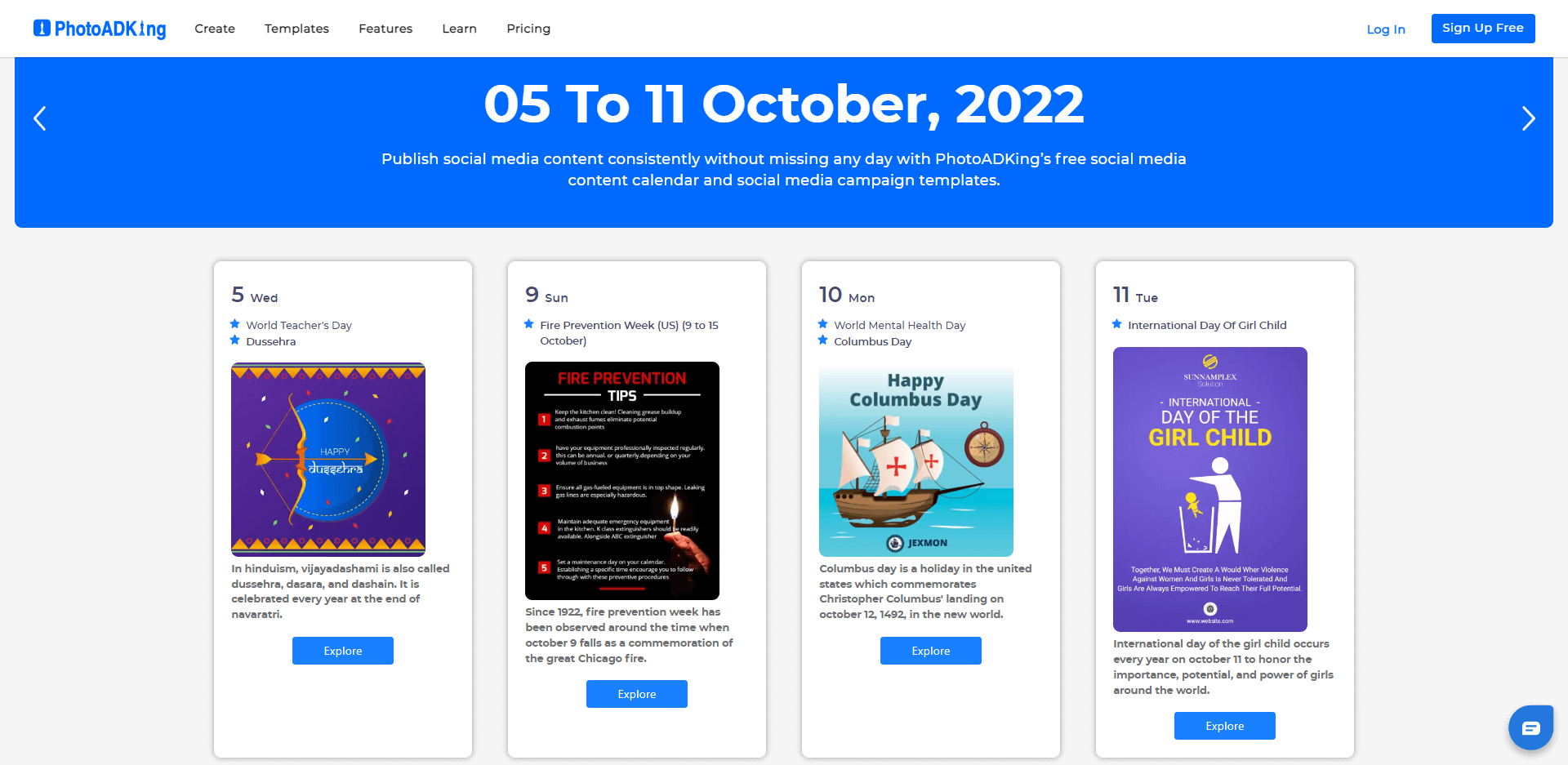**Desktop Screenshot of Photo AD King's Social Media Content Calendar**

The desktop screenshot showcases a section of the Photo AD King platform, which appears to be a comprehensive tool for managing and creating social media content. At the top-left corner, there is a small icon resembling an award, similar to an Academy or Oscar award, featuring a human figure and indicating it is associated with Photo AD King.

The navigation bar at the top features several options: "Create," "Templates," "Features," "Learn," and "Pricing." Additionally, there are buttons on the top-right for "Log In" or "Sign Up for Free."

The main content displayed on the screen promotes a social media content calendar for the week of October 5th to October 11th, 2022, offering templates to help users publish consistent content across their social media platforms. Highlights from the calendar include:

- **Wednesday, October 5th:**
  - **World Teachers Day** and **Vijayadashami (also known as Dussehra, Dasara, and Dashain)**.
  - An image accompanies these events showing an arrow piercing a circle.
  - Explanation: Vijayadashami is a significant Hindu festival celebrated at the end of Navaratri.

- **Sunday, October 9th:**
  - **Fire Prevention Week** in the U.S. (October 9th to 15th).
  - Listed fire prevention tips include maintaining kitchen cleanliness, regular professional equipment inspections, ensuring the safety of gas fuel equipment, having adequate emergency supplies, especially K-class extinguishers, and scheduling maintenance days.
  - A photo depicts someone holding a lit match, referencing Fire Prevention Week and its historic commemoration of the Great Chicago Fire since 1922.

- **Monday, October 10th:**
  - **World Mental Health Day** and **Columbus Day** (also known as Indigenous People's Day).
  - The visual shows an old ship with a compass.
  - Background: Columbus Day marks Christopher Columbus's landing in the New World on October 12, 1492.

- **Tuesday, October 11th:**
  - **International Day of the Girl Child.**
  - A purple poster displays a white cartoon character throwing a yellow baby into a trash can with a message advocating for violence-free environments and empowerment for girls.
  - Significance: This day honors the importance, potential, and power of girls worldwide, aiming to create a world where violence against them is not tolerated.

This section of the Photo AD King platform essentially presents an organized view of upcoming social media content, providing templates and ideas for consistent posting aligned with various global events.